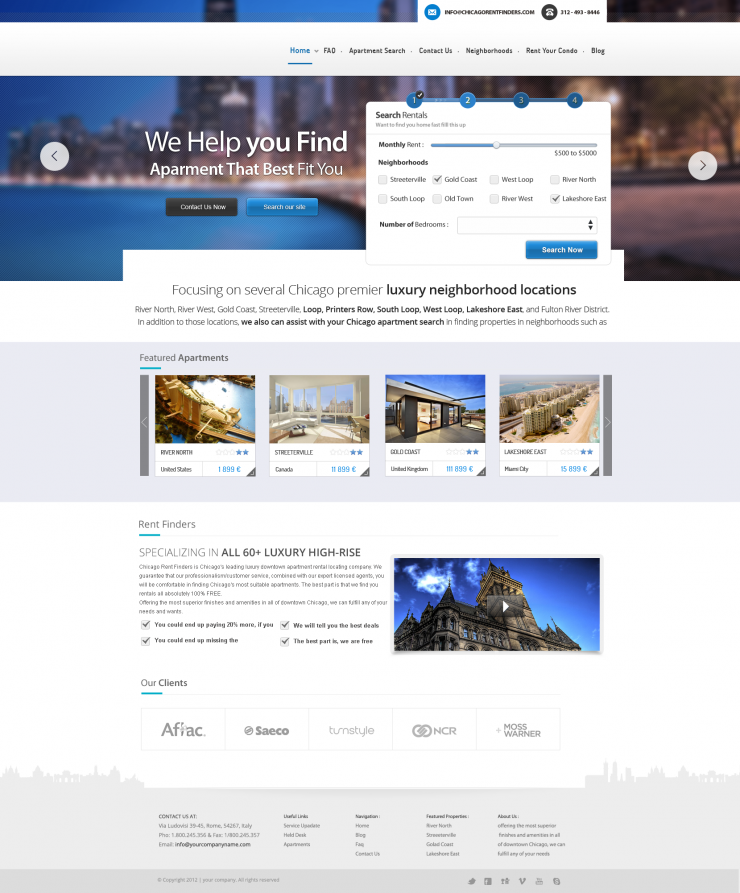Explore our website to find premier luxury apartments in Chicago's most sought-after neighborhoods! We specialize in high-end rentals in the Loop, Printer's Row, South Loop, West Loop, and Lakeshore East. Our expert team can help you with all your Chicago apartment search needs, ensuring you find the perfect home. We proudly serve clients such as AFLAC, SAECO, Turnstile, NPR, and Moss Warner. With our extensive knowledge and personalized service, we make finding your dream apartment easy and efficient. Contact us now to start your search for the ideal luxury condo in one of Chicago's premier high-rise buildings.